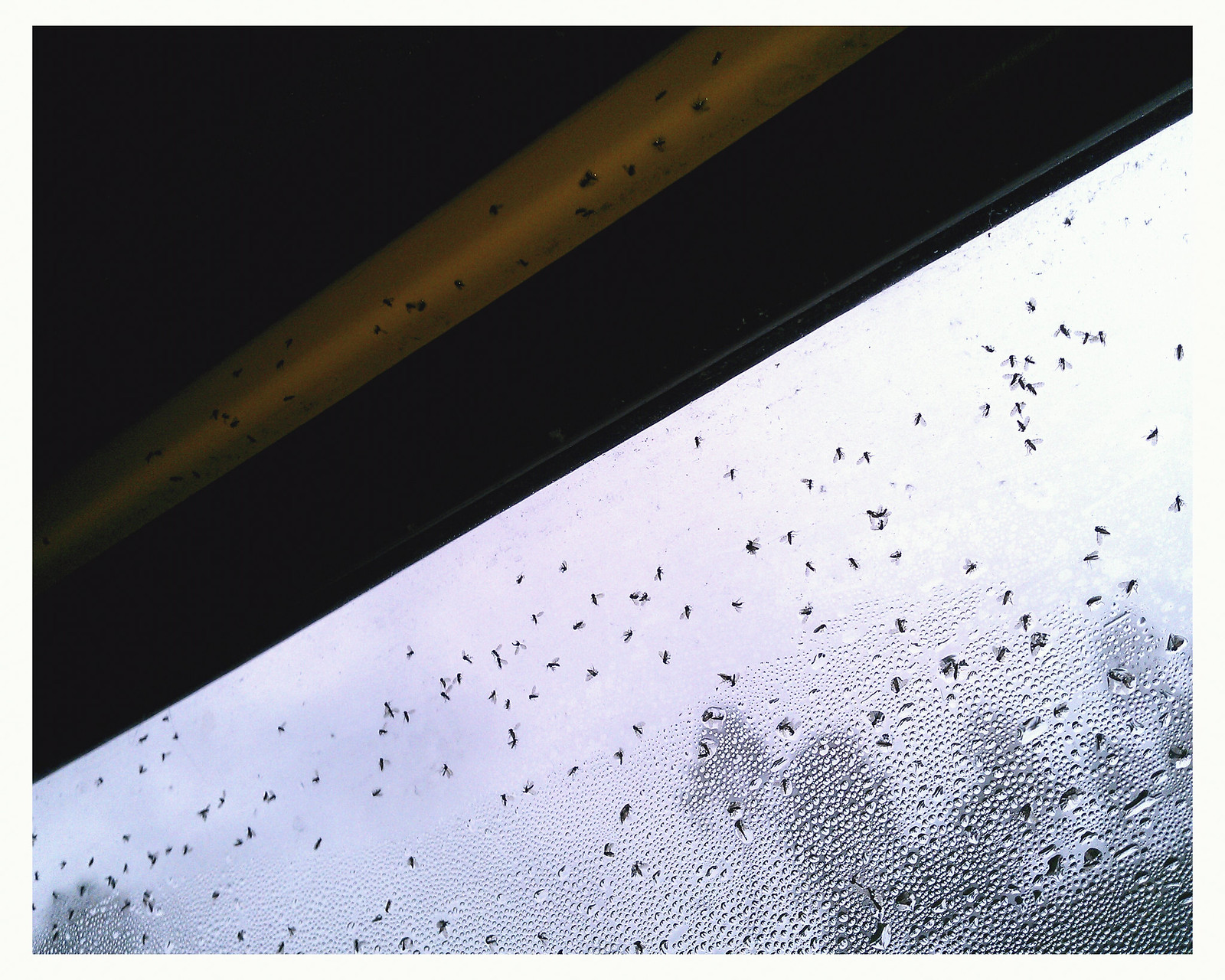This close-up photograph features a diagonal division of two contrasting materials that create an intriguing visual composition. On the bottom left to the upper right, a translucent surface, which appears to be glass with condensation or water droplets, dominates. This surface is dotted with numerous tiny black bugs, likely flies, scattered across it. The condensation adds a textured, almost misty quality to the glass, which has a bright sky and vague silhouettes of trees visible in the background, rendered fuzzy by the blue tint of the glass.

The upper left portion of the photograph, separated by a pronounced yellowish strip, displays a dark brown or reddish cylindrical pipe running from the left center edge to the upper right center. This pipe, too, is speckled with black bugs. The combination of the reddish cylinder and the white lower material, both infested with these tiny insects, creates a stark contrast against the overall brightness of the scene behind the glass. This interplay of textures, colors, and forms, amplified by the presence of the black bugs, creates a compelling and richly detailed image.